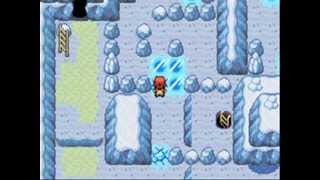The image appears to be a clear, color screenshot from an old top-down view video game, possibly a Pokemon game for a Game Boy console. The rectangular horizontal frame is bordered by narrow black strips on the left and right edges. Dominating the frame is a pale blue digital scene, depicting an intricate ice cave labyrinth with darker blue walls. The icy maze features crystalline shapes and pathways, with ladders located in the top left and bottom right corners. At the center of the scene is a cartoon character—likely a cat—with an orange-red head and a yellow body, navigating through the maze. The overall setting is bright, clear, and well-lit, with pathways marked by ice-covered floors and impassable white hills.